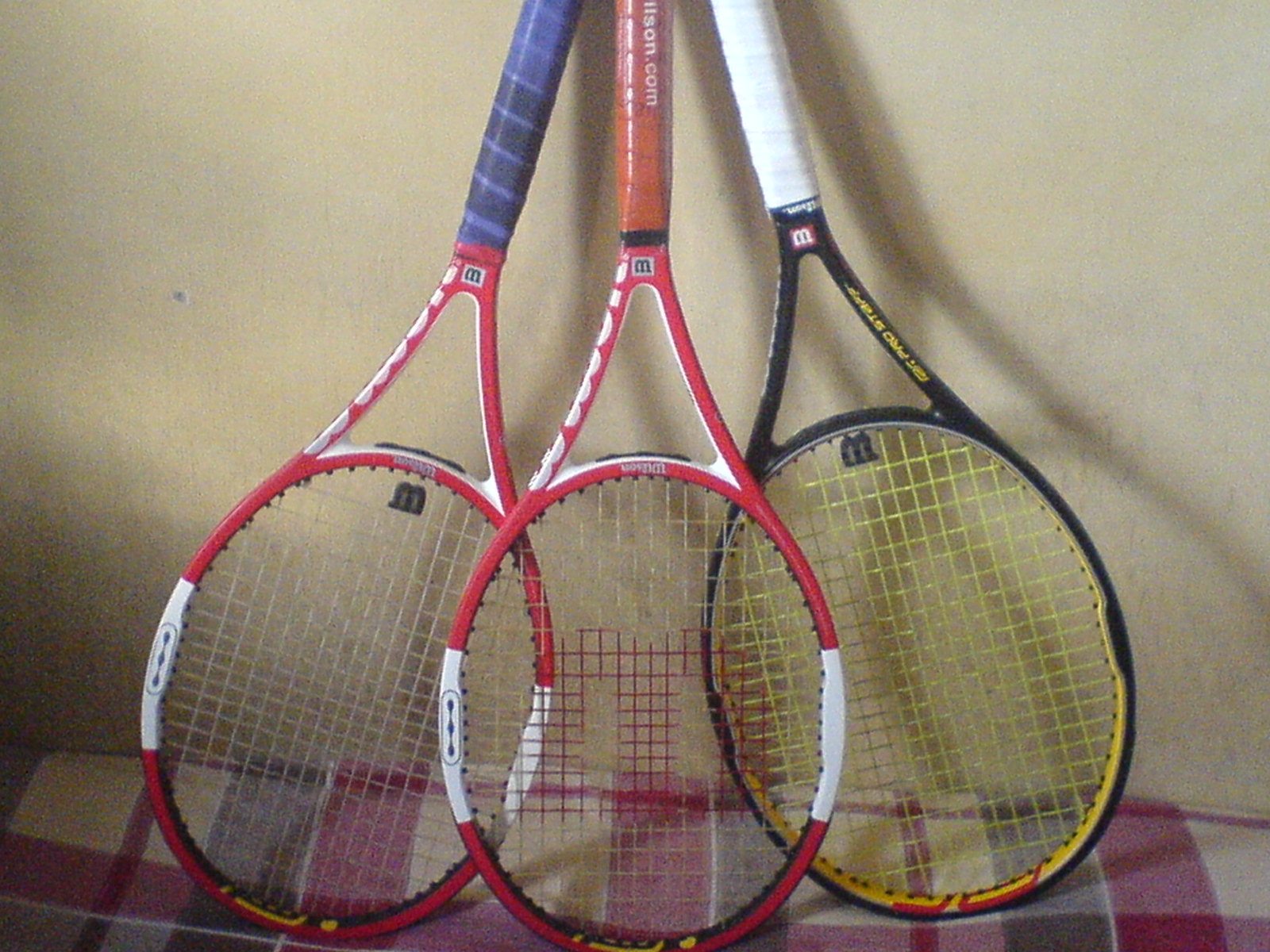This close-up photograph showcases three Wilson tennis rackets leaning against a light beige wall, their handles resting on the wall while the racket heads touch a plaid blanket that features stripes in red, dark gray, and beige. All three rackets share an oval frame design with a distinctive V-shaped throat where two pieces of metal converge into the oval. The racket on the left has a dark blue handle with black or dark purple stripes and is strung with whitish-yellow strings, featuring a small black "W" at the bottom. The middle racket, which appears in front of the other two, has a red handle with white writing that reads "Wilson.com" and is strung with yellow strings that also display a black "W" at the bottom. The racket on the right has a white handle, black oval frame with yellow interior accents, and is strung with yellow mesh, marked by a white "W" in a red rectangle at the bottom. The two rackets with red frames feature small black Ws in silver rectangles closer to the handles. All three rackets, detailed and distinct, share a common brand yet display varying colors and designs, resting against the soft palette of the room's decor.